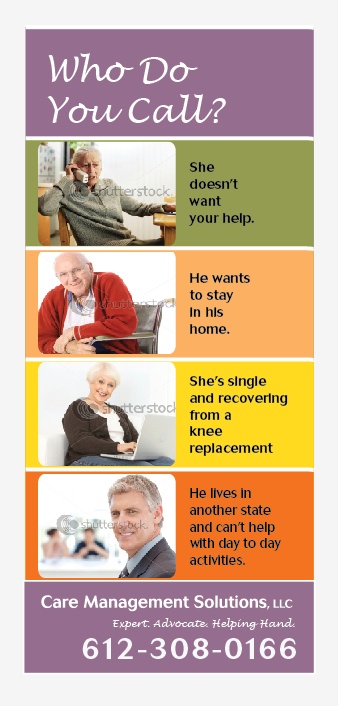The image depicts an advertisement for "Care Management Solutions, LLC" designed to offer support for elderly individuals. The ad is laid out in six distinct horizontal panels against a gray surface. The top panel is light purple with white text that asks, "Who do you call?" Below it, the second panel features a green background with an older woman talking on a phone, overlaid with black text stating, "She doesn't want your help." The third panel has an orange background and shows an elderly man in a red sweater smiling from a wheelchair, with the text, "He wants to stay in his home." The fourth panel, which is yellow, presents a short-haired older woman wearing a white top and brown sweater, using a laptop, accompanied by the text, "She's single and recovering from a knee replacement." The fifth panel, in orange, features a middle-aged man in a business suit smiling, with the words, "He lives in another state and can't help with day-to-day activities." All images bear the watermark "Shutterstock." The final panel is light purple again and includes the company name "Care Management Solutions, LLC," along with the phrase "Expert, Advocate, Helping Hand," and the contact number 612-308-0166 in white text.